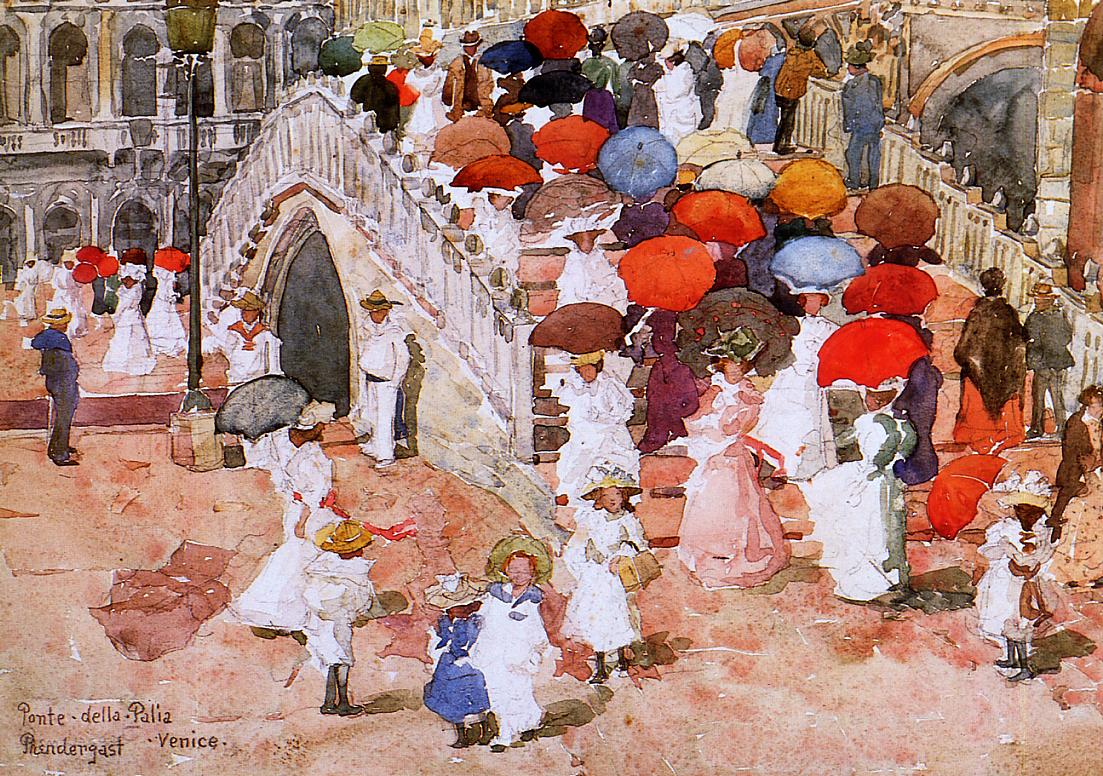This is a vibrant watercolor painting with a post-impressionist style, capturing the bustling scene on and around the Ponte della Paglia in Venice, Italy. The arched bridge stretches over a serene canal, with its tunnel visible underneath. Brightly colored umbrellas—red, blue, orange, and more—dot the landscape, held by numerous figures walking across the bridge. Most of these figures are women in white dresses, though some are in black or red, and a few men in hats also feature prominently. The scene includes children playing by the canal, also adorned in dresses and sun hats. The vibrant, colorful umbrellas and varied attire bring a lively energy to the image, which is further enhanced by decorative columns, doorways in the background, and a classic light post beside the bridge. The lower left corner of the painting is inscribed with "Ponte della Paglia, Venice," affirming the Italian setting.